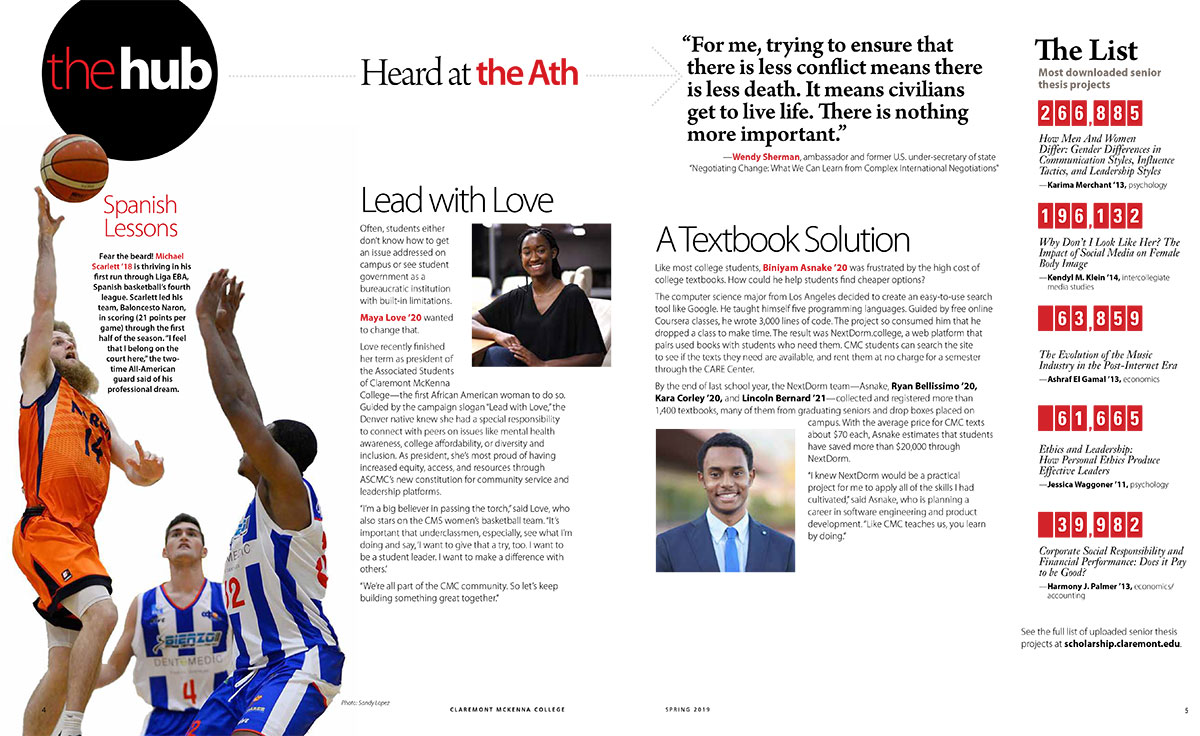In this image, we see a vibrant, text-laden page showcasing various sections dedicated to different topics. At the top left corner, the heading reads "Spanish Lessons," drawing the eye with its compelling font. Below this heading, a subheader boldly states, "Fear the Bird," setting a dynamic tone for the content that follows.

The main body of the text highlights the impressive achievements of Michael Scarlett, an 18-year-old thriving in his debut season in Liga EBA, Spain's fourth-tier basketball league. Scarlett is lauded for leading his team, Baloncesto Naran, with an average of 21 points per game through the first half of the season. His quote, "I feel that I belong on the court here. It took time," reflects his dedication and the fulfillment of his professional dream, despite the inherent challenges.

Accompanying this sports narrative, the page touches on the struggles and aspirations of students within academic and bureaucratic settings. An observation is made about how many students either lack the knowledge to address issues on campus or perceive student government as a limited, bureaucratic entity. 

Among these narratives is also the story of Miniyam Ashnake, a 20-year-old who, like many college students, was frustrated with the high cost of textbooks. The text hints at Ashnake's efforts to find more affordable solutions for students, emphasizing the proactive stance young individuals are taking to solve common problems.